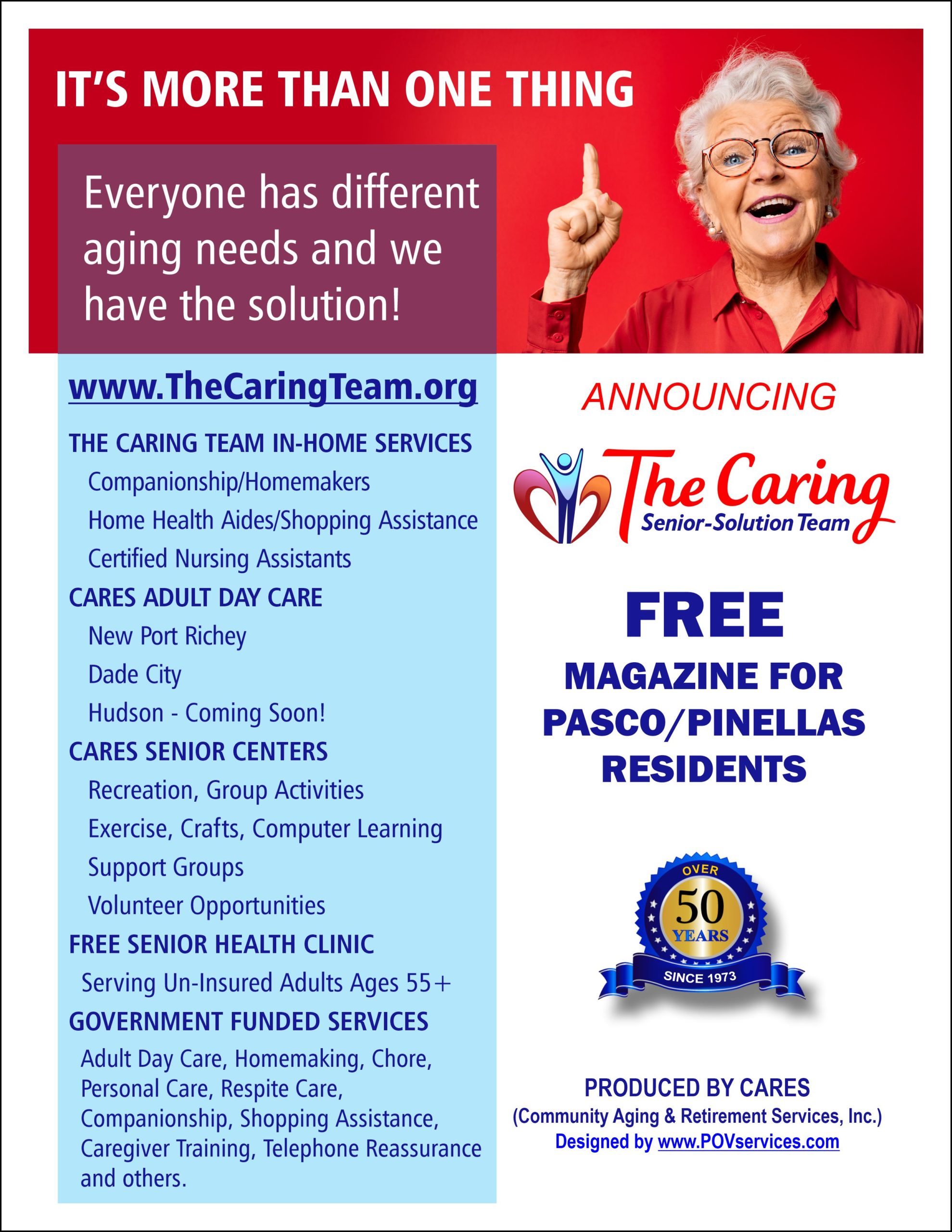This flyer is designed in a rectangular, portrait layout. At the top, a bold headline in white font reads, "It's More Than One Thing," set against a vibrant red background. Just below this text, an older lady is featured against the same red background, pointing upwards to draw attention to the message. The flyer continues with the statement, "Everyone has different aging needs. We have the solution," emphasizing the range of services offered.

The name of the company, "Caring Senior Solution Team," is prominently displayed. The flyer also highlights a special offer: "Free Magazine for PASCO/Pinellas Residents." 

On the left-hand side, detailed information about the various services provided by the company is listed in blue font against a light blue background, providing a clear and organized overview. 

A noticeable symbol on the right-hand side proudly states, "Over 50 Years," indicating the company’s extensive experience in the field.